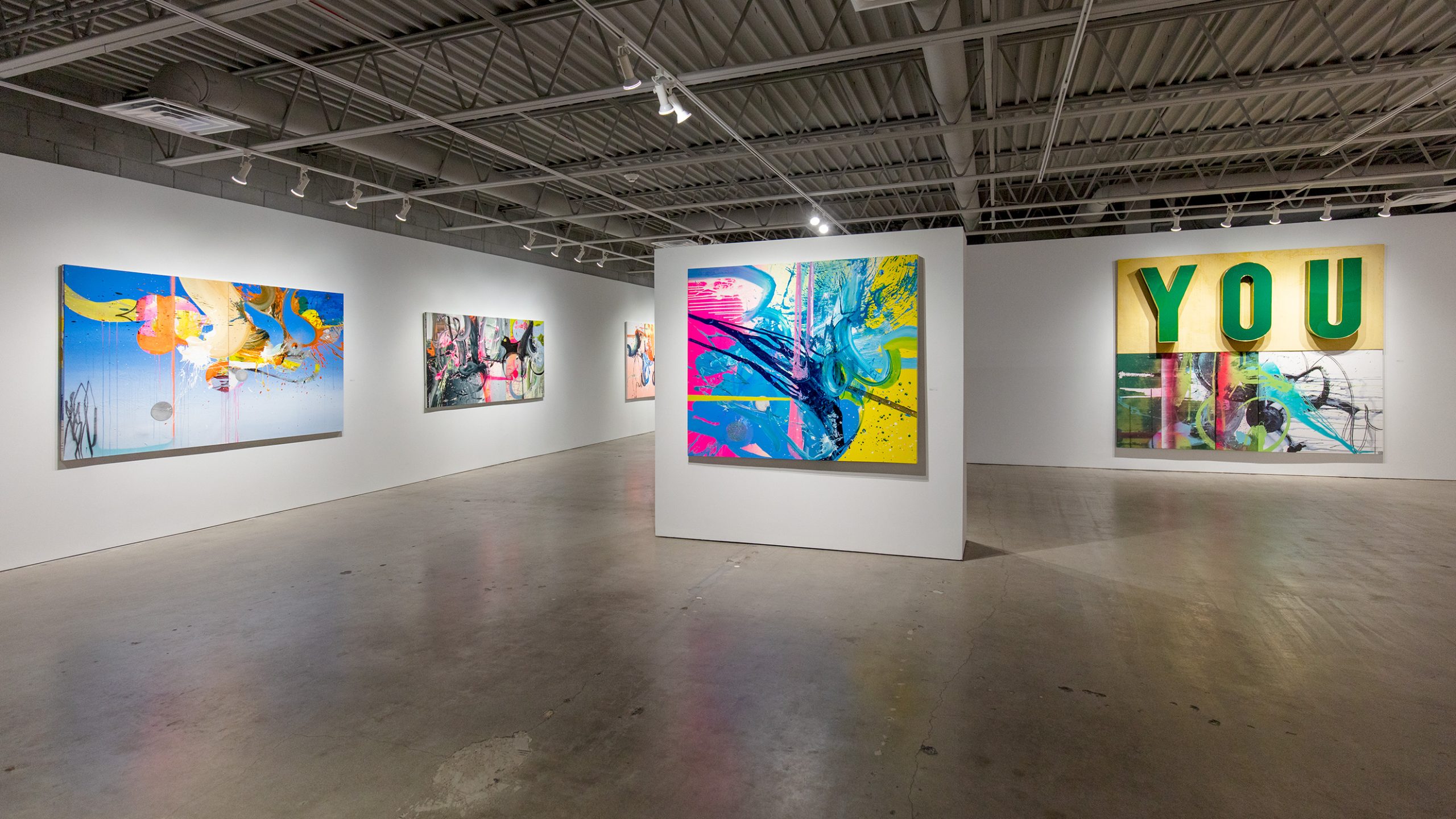The photograph captures a spacious art gallery set in a large warehouse. The warehouse features a high, metallic ceiling with grates and rows of overhead lights of a flashlight design. The floor is made of grey stone, giving the space an industrial aesthetic. Dominating the left side of the gallery are three large paintings displayed on the far wall. The central piece on this wall is an abstract artwork with vividly tossed splashes of paint, including a dramatic black splash in the middle, surrounded by pink and blue, suggesting a random yet expressive pour of paint. Adjacent to it, an artwork prominently features the letters "Y.O.U" in green, with an abstract paint splash beneath it.

In the middle of the spacious room stands a solitary dividing wall, resembling an island, showcasing a large canvas. This artwork is rich in bright colors, including light blue, pink, yellow, and black, characterized by its dynamic and chaotic abstract style. Against the right wall, another notable piece continues the vibrant and abstract theme, adding to the cohesive yet eclectic display of the gallery. The white walls and minimal furnishings ensure that the vivid art pieces remain the focal point, while the architectural elements of the warehouse space add to the modern and unconventional atmosphere of the exhibit.